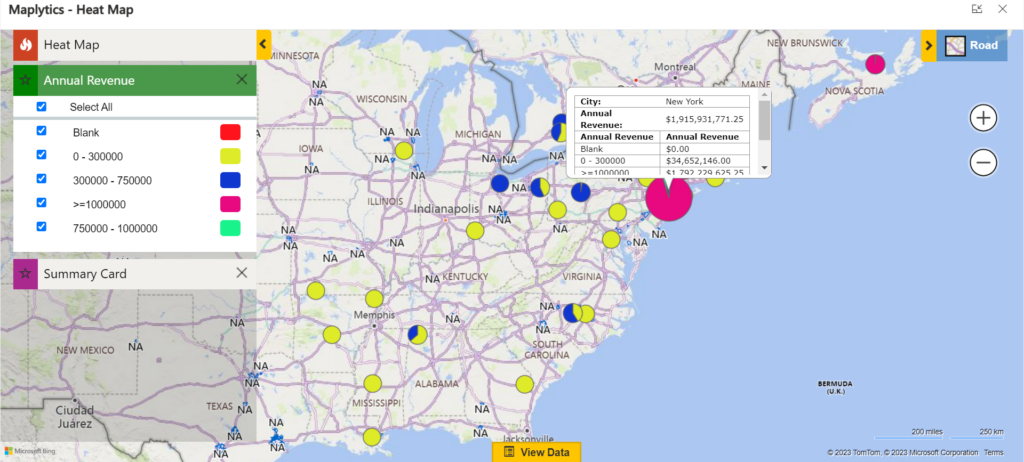This is a comprehensive description of a heatmap using the Maplytics application, depicting various data points related to annual revenue across the United States. The interface displays the following:

At the top, the title "Maplytics-Heatmap" is prominently featured. Below this header, the main section of the image showcases a map of the United States with the Atlantic Ocean visible on the right-hand side.

On the left-hand side, an overlay box affecting the map content is visible. The box starts with a heading labeled "Heatmap." Directly beneath this, a green bar indicates the filter criterion "Annual Revenue."

Following this heading, a selection menu, initiated with "Select All," is outlined. The color coding within this menu includes:
- A red box associated with "Blank" entries.
- Yellow signifies entries ranging from "$0 to $300,000."
- Blue indicates figures between "$300,000 to $7,500,000."
- Pink denotes entries exceeding "$100,000."
- Green applies to the range "$7,500,000 to $1,000,000."

Further down, another banner labeled "Summary Card" features a purple box accompanied by a star icon.

The map itself is dotted with circles of various colors representing different data points. These circles vary in color:
- Predominantly yellow circles.
- Mixed yellow and blue circles.
- Isolated pink circles, alongside a larger pink circle with a section removed.

The larger pink circle, in particular, appears to highlight a specific area—possibly New York City—as part of the depicted data.